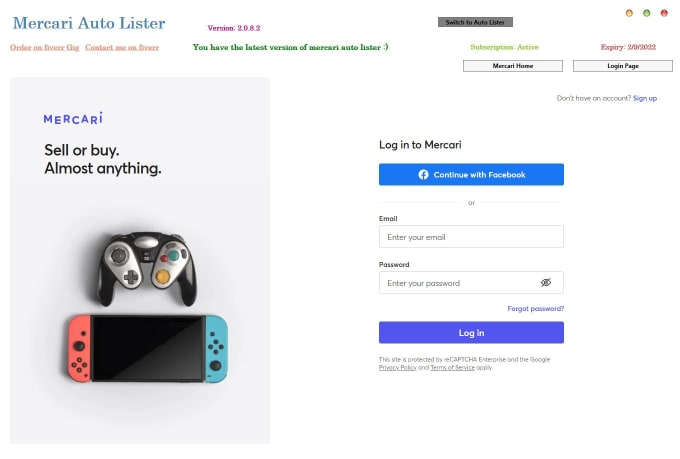**Image Description:**

The background of the image is light gray with a dark blue gradient at the top where the word "Makkari" is prominently displayed. Below "Makkari," the text "Sell or buy almost anything" is written in black. Centered in the middle of the image is a black video game controller featuring a silver tab in the middle and two silver extensions on either side. The left extension includes a directional pad, while the right extension is populated with buttons: a green button, a red button, a yellow button, and two black buttons.

Beneath the controller is a miniature tablet, distinguished by a pink section on the left side and a blue section on the right side, each section containing a series of holes which could either be for speakers or buttons. Additionally, there is a prominent button on each side of the tablet. To the left of this tablet and beneath the controller, shadows cast on the surface below are visible, adding depth to the layout.